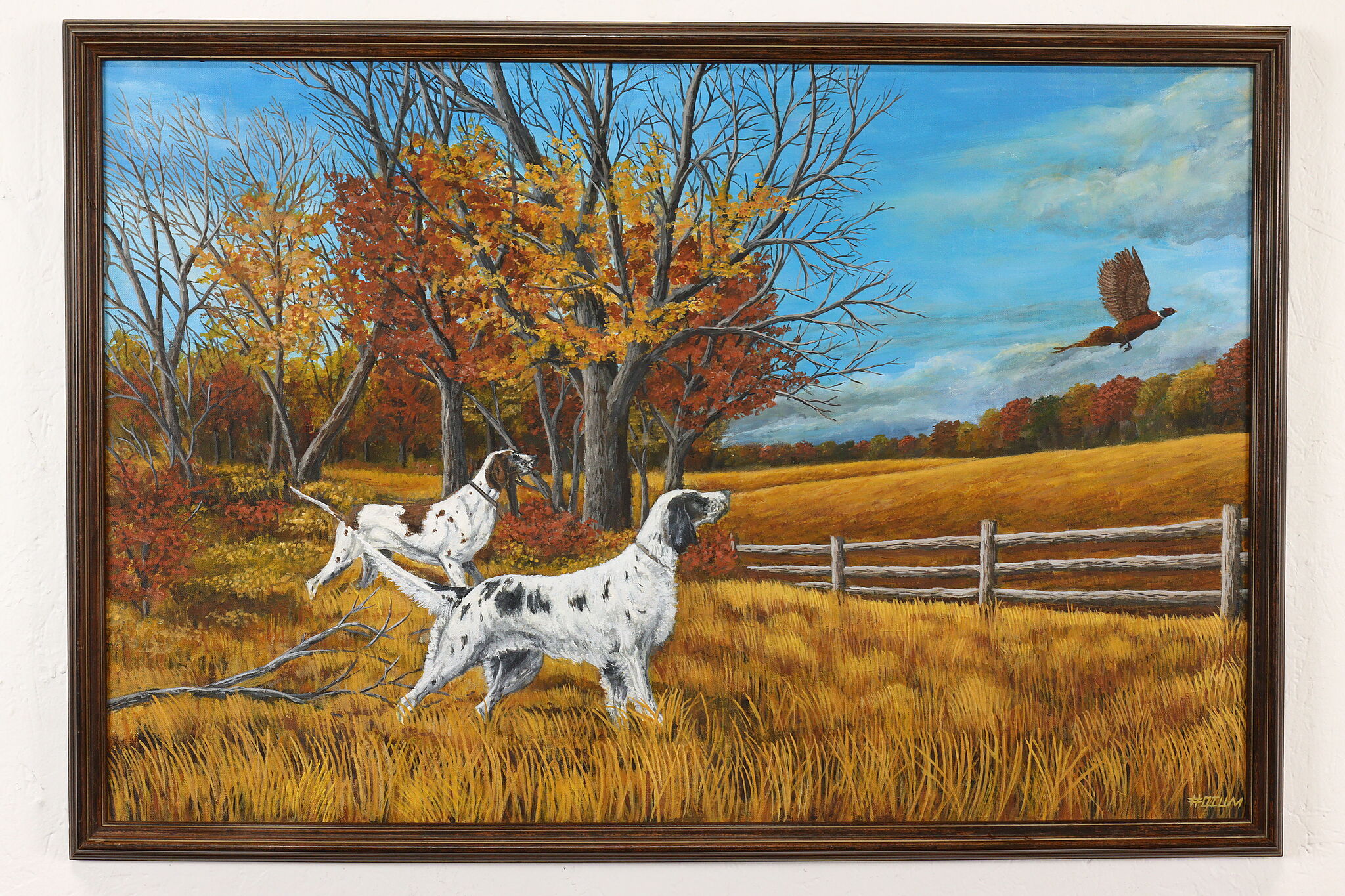In this detailed painting set in an autumnal countryside, two white springer spaniels, one with brown splotches on the left and the other with black splotches on the right, are captured staring intently at a brown pheasant with large wings as it takes flight. They stand in a golden, straw-like field that stretches endlessly into the horizon. The dogs' alert, pointed tails suggest their focus and training as hunting dogs. Surrounding the scene, a plethora of vivid, colorful trees — boasting reds, yellows, and greens amidst their mostly barren branches — populate the background, indicating the vibrant, yet dying foliage of autumn. Some trees are starkly bare, with detailed brown trunks visible, and a wooden fence runs distantly through the scene. The sky above is a crisp blue with fluffy white clouds, further enhancing the outdoor, seasonal atmosphere. In the bottom right-hand corner, the artist's signature marks the piece, accentuating its crafted authenticity.